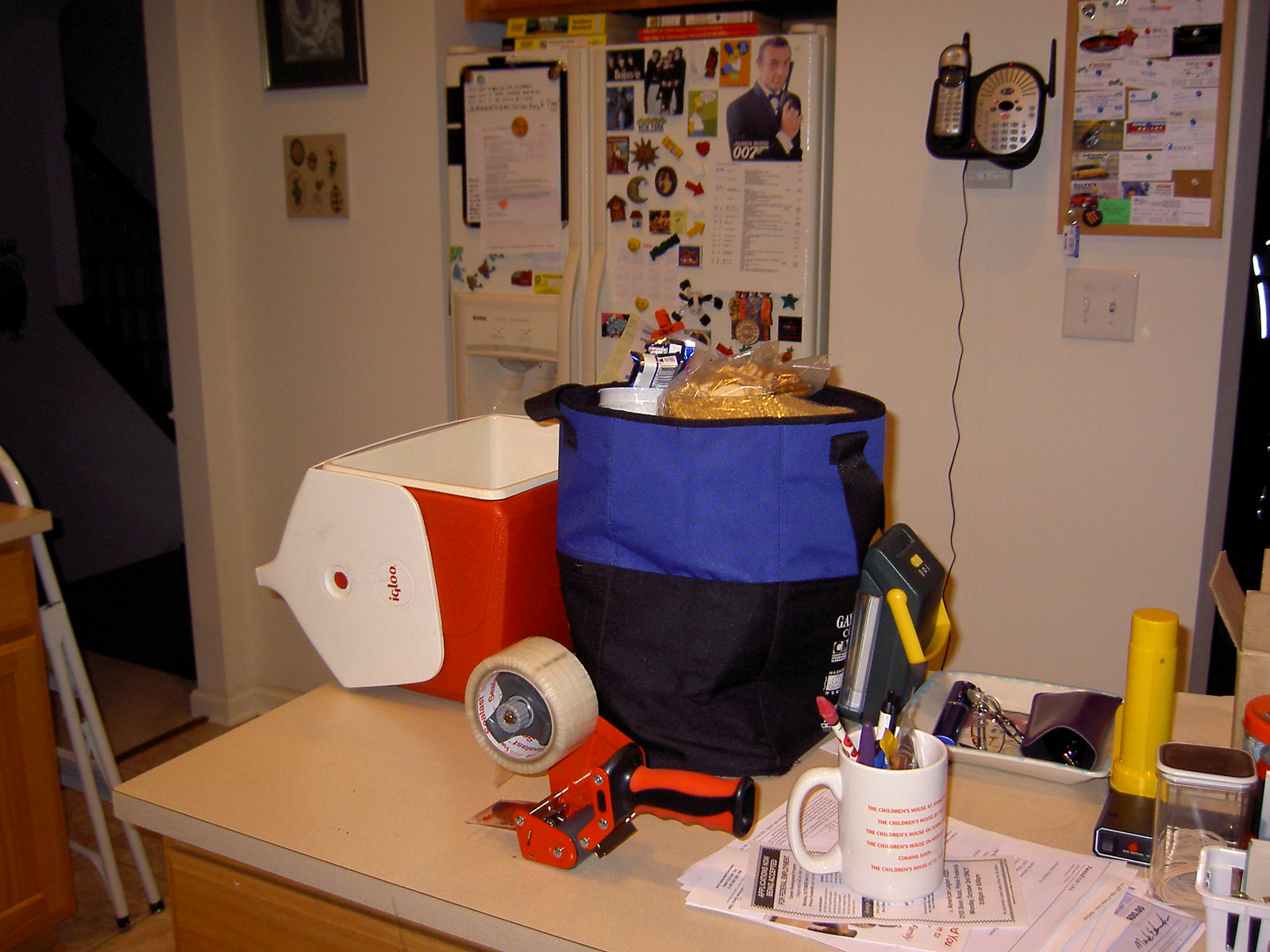The image depicts a busy kitchen scene packed with various items and details. The kitchen walls are adorned with several framed pictures, although they are too distant to make out clearly. The focal point is an older model white refrigerator equipped with an ice maker. The top left door of the fridge features a to-do list, while the right door is festooned with an assortment of magnets, including pop culture references and a notable 007 James Bond magnet. A grocery list is also visible on the right door.

Adjacent to the refrigerator on the right, a cordless phone charging base is wall-mounted, the base itself doubling as a phone with a visible dialing pad. Further right, a corkboard brimming with business cards, push pins, and other notes hangs on the wall. Beneath the corkboard, there are two light switches, with one currently in the on position.

On the left side of the image, part of a kitchen counter is visible, featuring a gray step stool and a partial view into another room. Dominating the foreground is a white countertop cluttered with various items: an open red and white Igloo cooler, appearing empty; a blue and black tote bag containing grocery items like bread and snacks; a large roll of mailing tape on a dispenser, commonly used by movers; a white mug with indecipherable red lettering filled with pens; and several pieces of mail and billing statements.

A white tray sitting on the counter holds a collection of personal items, including lipstick, eyeglasses, an eyeglasses holder, and a yellow flashlight. Nearby rests an old-style alarm clock, and a black device with a yellow handle that resembles a vintage coin dispenser used in meter maids or fast-food restaurants. The scene captures a snapshot of everyday life, rich with the diverse, utilitarian objects that inhabit this lived-in kitchen.